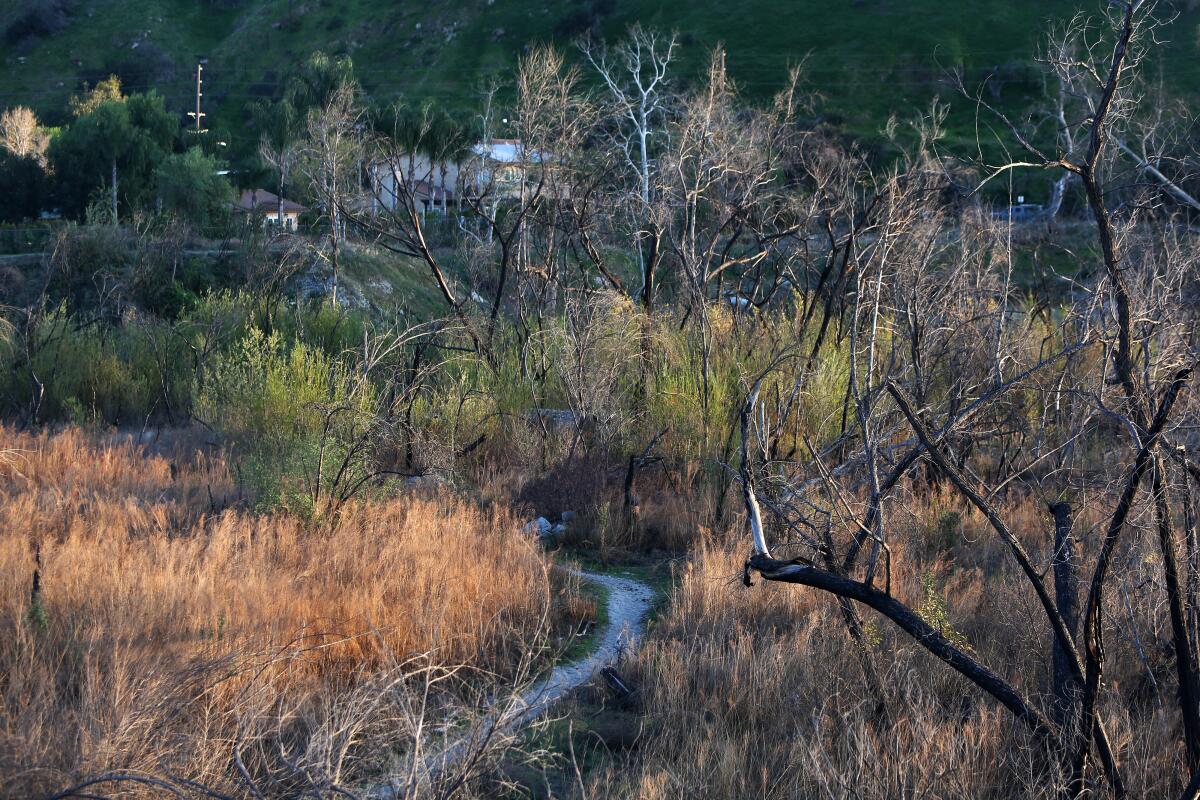The image captures a sunlit woodland scene, likely during late fall or winter. The foreground features numerous tall trees with bare branches, and the ground is covered in tall, tan-colored weeds interspersed with shorter, green bushes. A meandering dirt footpath snakes through the center of the image, leading towards a more densely wooded background. Amidst the trees, glimpses of white buildings can be seen, partially obscured by the branches. The middle ground transitions into a green hillside, and a car is visible on a distant road. The setting is illuminated with bright, natural daylight, highlighting the contrast between the brown, lifeless elements in the foreground and the greener areas further back. This picturesque outdoor scene is devoid of any textual distractions, allowing the viewer to fully immerse in its rustic beauty.